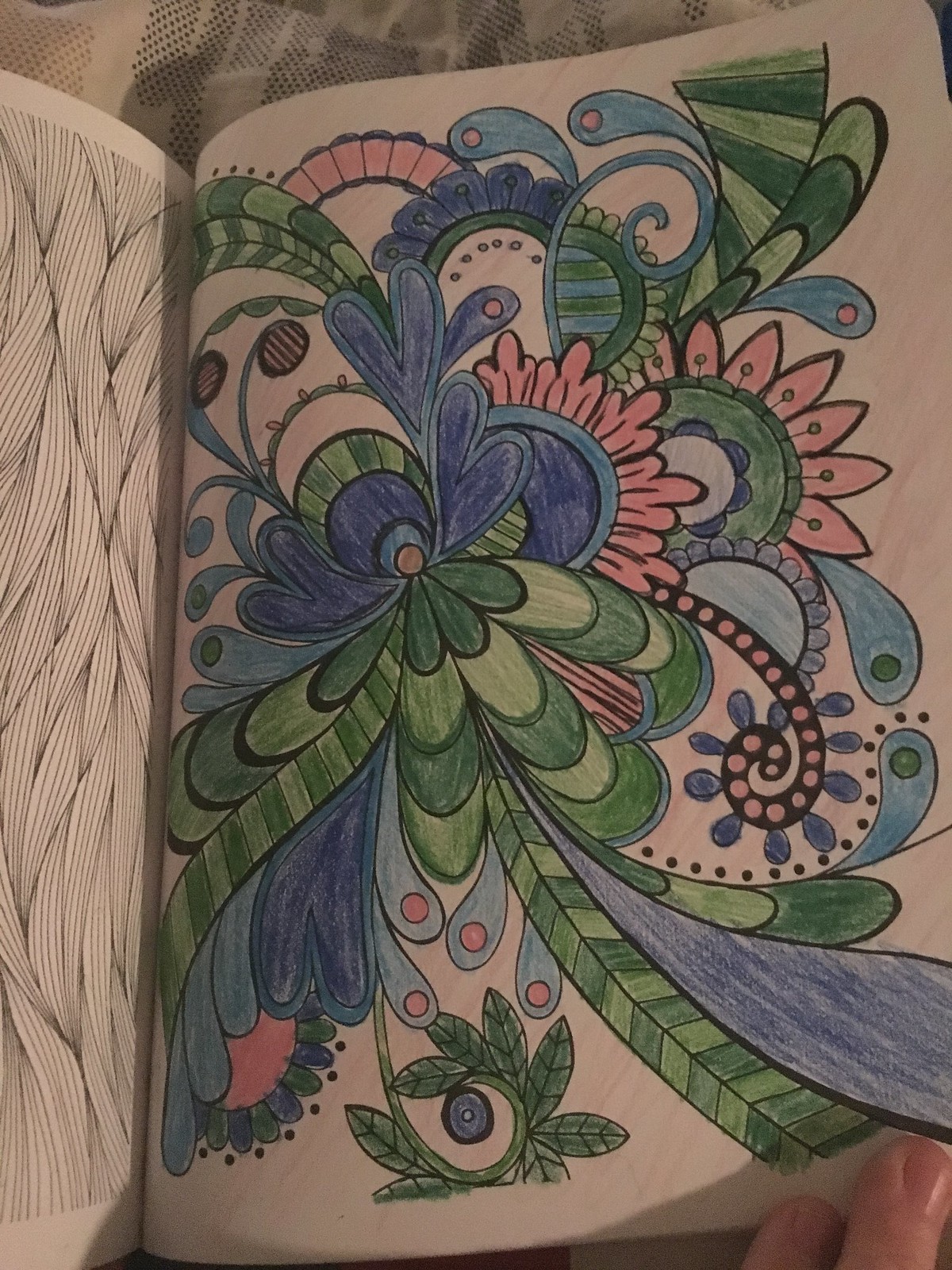This is a detailed photograph of a coloring book page, showcasing a vibrant and intricately colored design. The primary motif is a large, spirally flower with an array of petals and leaf-like shapes extending outward from the center. The petals and leaves are filled in with a rich palette of dark and light greens, blues, light blues, purples, and pinks. The flower features large, rounded green and dark green petals, alongside long, heart-like blue petals. There are also feathery blue and pink petals, pointy pink petals, and a swirl of small green leaves with a blue circle at their center. The background of the coloring book is white, with the left side displaying rope-like spiral designs in black and white, though only half the page is visible due to the left margin of the photo. In the bottom right corner, two fingers are holding the book open against a white, linen-like tablecloth that serves as the backdrop of the photo. The overall feel is of a carefully colored, pre-drawn sketch in a sketchbook, with the colors meticulously applied to bring the intricate floral design to life.